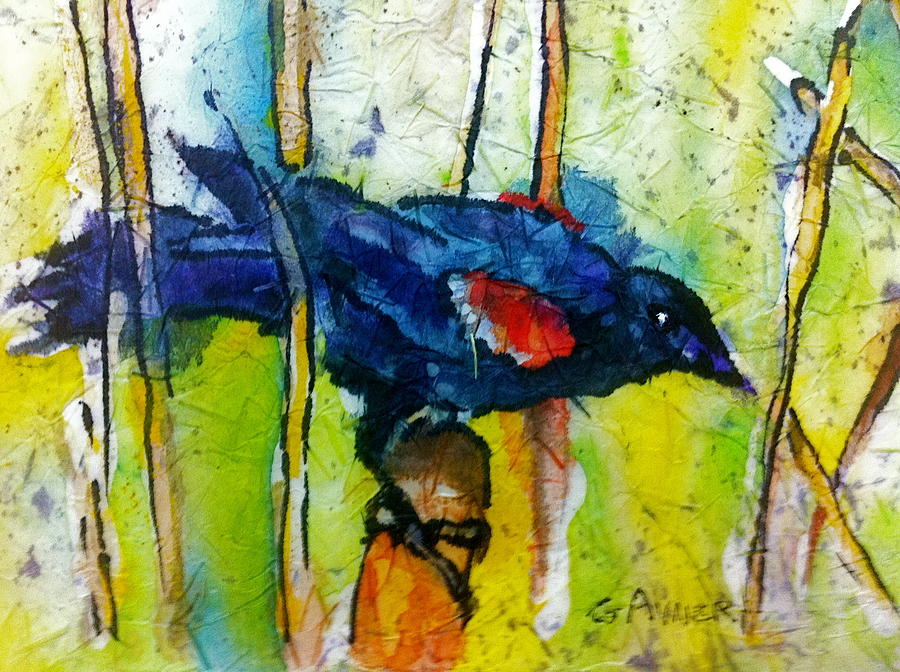This piece of artwork is a detailed watercolor painting of a vibrant blue bird with distinct black talons and a small red patch on its wings. The bird is perched on a wooden structure, surrounded by an assortment of sticks. Created on a textured, slightly wrinkled surface, the background features a white base adorned with subtle green, yellow, and light blue splatters, along with vertical yellow strips. Additionally, a small signature is present at the bottom of the piece, adding a touch of authenticity to the captivating scene.